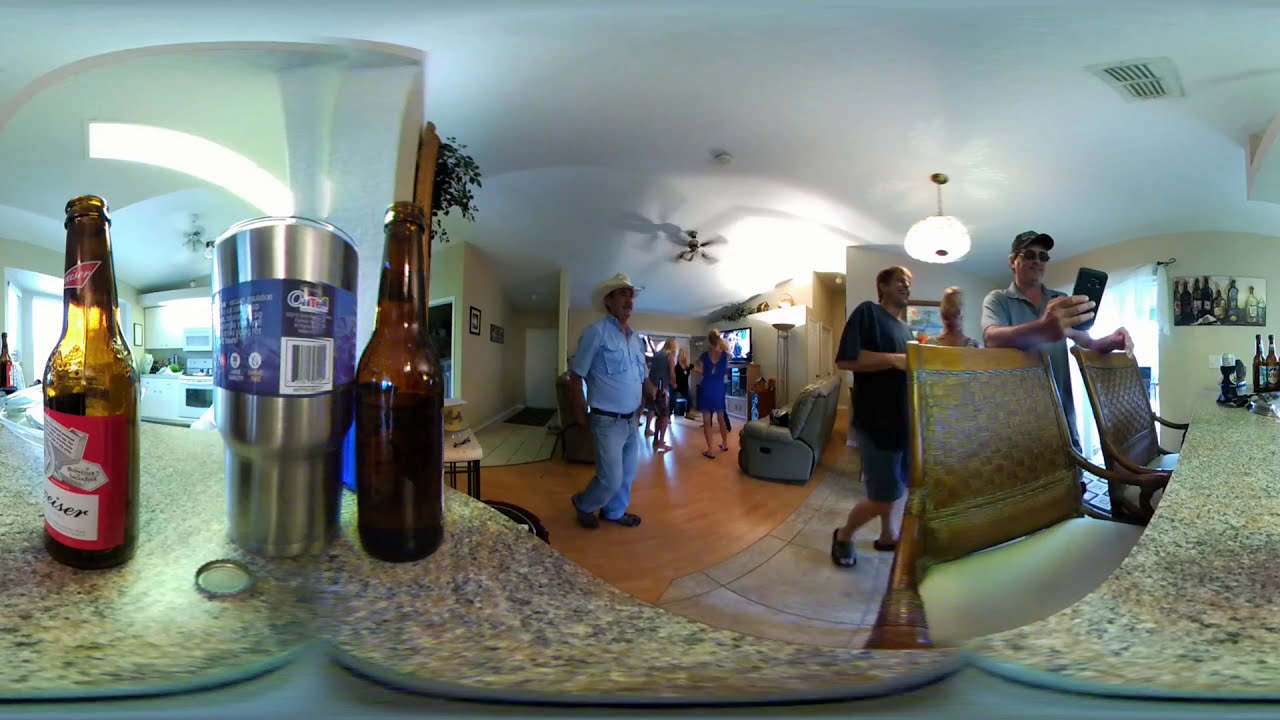This image captures a lively indoor party scene in someone's living room, which features white walls and ceiling, complete with an overhead fan. The setting is cozy yet spacious, with wooden floors and what appears to be a large, slightly warped photo effect that loops the scene in a circular manner. In the foreground, a tan, black, and gold granite countertop displays two empty beer bottles—a Budweiser and another brown bottle—and a silver metal cocktail shaker. On the darker side of the countertop rests a beer cap. Two padded, armrest-equipped bar stools stand beside the counter, though unoccupied.

Central to the image is a well-depicted living area, showing a man in a black baseball hat and sunglasses, dressed in a gray shirt, who appears to be taking a selfie with his phone. Behind him, another man wearing a black t-shirt and blue shorts just above his knees, along with brown leather sandals, approaches. A third gentleman, in the background, sports a denim shirt, Levi jeans, work boots, and a cowboy hat. Also visible is a floor torch light next to what might be a sofa or large easy chair.

The gathering is further evidenced by additional beer bottles and liquor visible on the side counter. Overall, this room, potentially part of a larger living and dining area, is buzzing with social activity and accentuated by various details such as the ceiling fan, floor light, and unique decor elements.